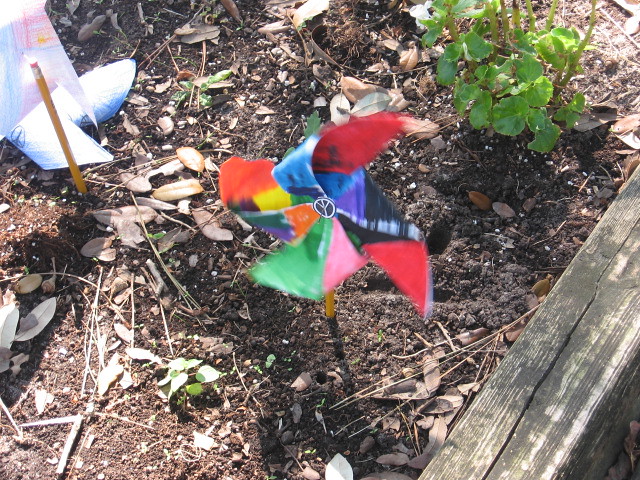In this photograph, a sunny day casts light and shadows over a raised garden bed, bordered by an old, weathered wooden plank. The garden bed, still early in its growing season, features a single small green plant with sprouts of leaves. In the soil, two yellow wooden pencils are stuck into the ground, each adorned with hand-crafted pinwheels made from light, colorful materials. The more prominent pinwheel, affixed to one pencil, showcases a vibrant patchwork of colors including orange, blue, red, purple, black, pink, green, and yellow. It has four spokes and a small black button with a white peace sign at its center. The second pencil, located farther to the left, holds another, somewhat disheveled pinwheel with pink and purple hues, parts of which have fallen to the ground. Both whimsical creations bring a touch of handmade charm to the nascent garden.